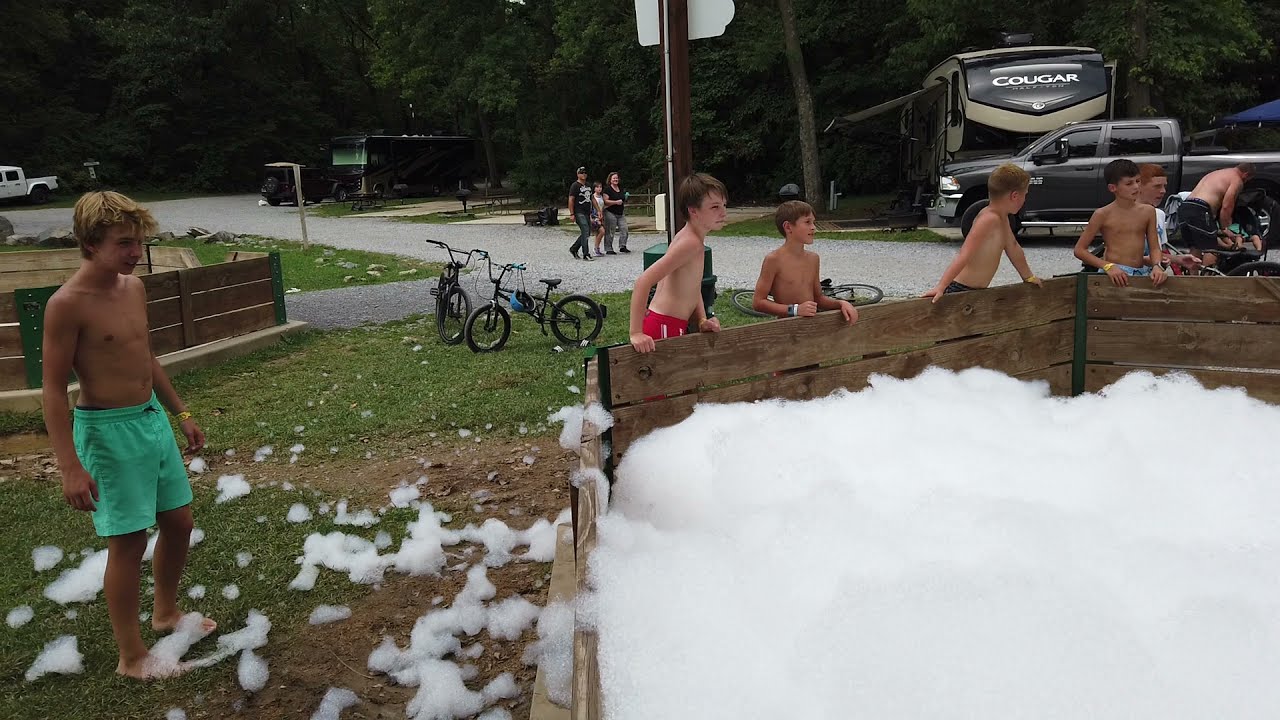In this lively outdoor scene, a group of about seven young boys, all wearing swimming shorts and no shirts, gather around an octagonal wooden fence enclosure filled with soapy bubbles. The bubbles spill onto the grass outside as well. The boys appear captivated as they look into the foamy area, suggesting some exciting activity is taking place inside the enclosure. To the left, one boy in turquoise aqua shorts stands out as he gazes into the foamy spectacle. The background features a gravel road with people walking, along with bicycles parked nearby. There are various vehicles, including a large white bus labeled "Cougar," a black truck, and another white truck further back. The setting hints at a recreational or event space, with street signs and several campers parked around, giving it a vibe akin to a campsite or a communal outdoor area in the southeastern United States.